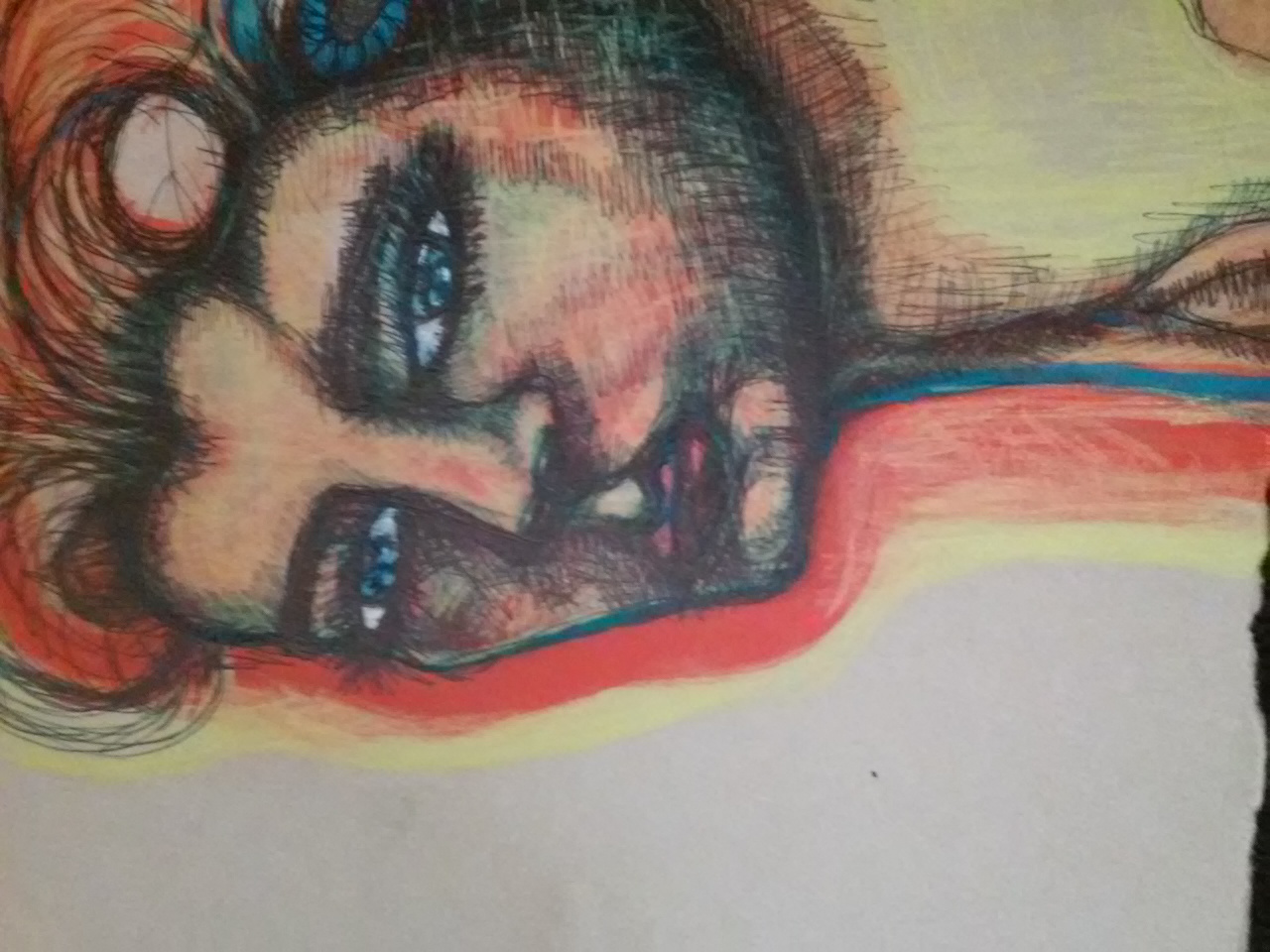The image is a detailed colored pencil drawing, slightly taller than it is wide, depicting a close-up of a person's head and neck against a white background. The figure, emerging from the right side of the frame, bears characteristics reminiscent of a Greek model. The skin tones are composed of nuanced shades of yellows, reds, and tans, with considerable black ink or pencil shading creating a dimensional effect. The person has wide, blue eyes set in a sad expression, a prominent nose, and pinkish lips. Their round face is framed by curly, almost red hair, highlighted with red and blue accents, possibly suggesting a perm. Their long neck, which is about as tall as their head, contributes to a stately yet delicate appearance. Notably, the person’s chin appears masculine, complete with an Adam's apple, blurring traditional gender lines. The canvas exhibits signs of wear, with some tearing visible on the bottom right and left edges. The left side of the face is surrounded by a red glow that extends down the neck, adding to the surreal, slightly cartoonish style reminiscent of "Duckman."